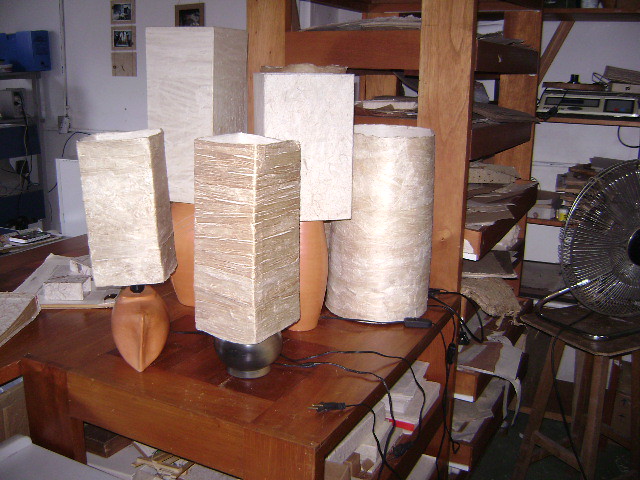The photograph depicts an indoor setting, likely a workshop or classroom, characterized by its organized clutter. Dominating the scene is a brown wooden table, upon which various lamps with different colored and shaped shades are displayed. The lamps' bases vary from a light tan terracotta to a dark gray, with some lamps obscured by others. In total, there are five lampshades, four of which are rectangular and one cylindrical, with varying hues of beige, tan, white, and light brown. 

One prominently features a light brown base resembling a shoe with a rectangular beige shade, while another has a chocolate brown vase-like base also with a rectangular shade. Papers spill out from an open drawer beneath the table, adding to the bustling ambiance. 

To the right, a brown wooden stool supports a metal fan, hinting at the room's functional nature. The background showcases white walls adorned with photographs and electronic devices, possibly industrial scales, housed on wooden cabinets with shelves. These shelves also display an array of materials, including carpets and other items. The entire setting suggests a space devoted to crafts or technical work, with an eclectic mix of utilitarian and decorative objects.